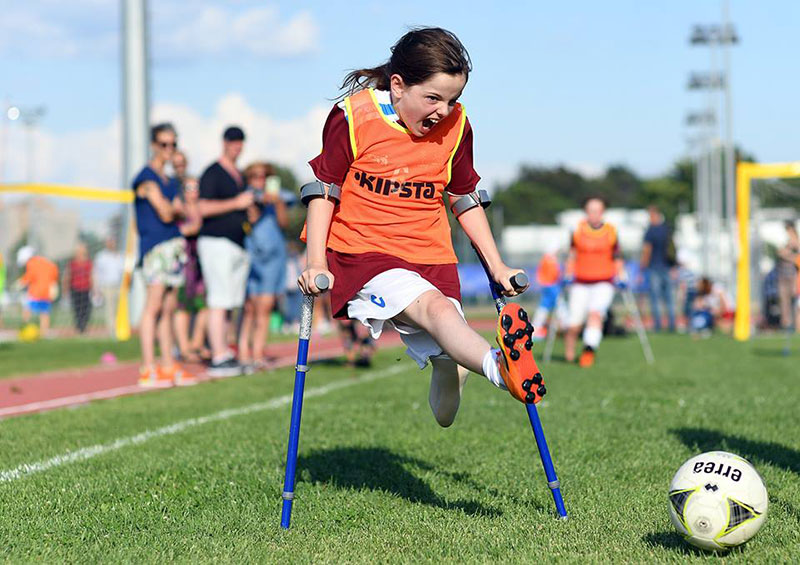In this vibrant color photograph, a young girl is captured in mid-action on a green grass field, participating in what appears to be a Paralympic or similar event for differently-abled individuals. The girl, who is an amputee with part of her left leg missing, is utilizing blue crutches that wrap around her arms, aiding her as she attempts to kick a soccer ball. She is dressed in an orange Kipsta jersey over a burgundy t-shirt, paired with white shorts. Her face is animated, with her mouth wide open, reflecting her determination and focus as she raises her leg to connect with the soccer ball, showcasing her black cleats with an orange sole. Surrounding her, the blurred background suggests spectators—possibly parents—watching and smiling at the touching moment. The scene is framed under a blue sky speckled with gray and white clouds, with green trees and a yellow-bordered goalpost visible in the distance, effectively illustrating a joyful and supportive environment.